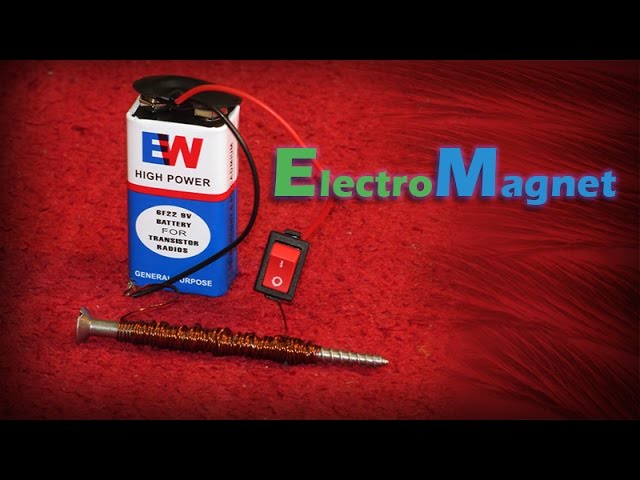The image is a well-aligned rectangular photograph featuring a detailed depiction of an electromagnet setup. It includes a thick black border at the top and bottom, and the central area showcases a dual-textured red surface: fine powder on the left and windblown sand on the right. Dominating the middle left of the composition is a vertically standing nine-volt rectangular battery by the EW brand, distinguished by its blue bottom, white top, and prominent "EW" initials—where the "E" is blue and the "W" is red—accompanied by the label "high power."

Connected to the battery are red and black wires, with the red wire extending towards the right and the black wire protruding towards the front. These wires link to a long screw wrapped in fine copper wire, situated near the battery. To the right of the battery, the word "Electromagnet" is prominently displayed, with "Electro" in green block letters and "Magnet" in blue block letters against the red backdrop. An on/off switch, encased in black with standard "1" and "0" indicators, is also part of the setup, and currently positioned in the off state. This image effectively illustrates the components and assembly of an electromagnet, providing a clear example of its structure and function.